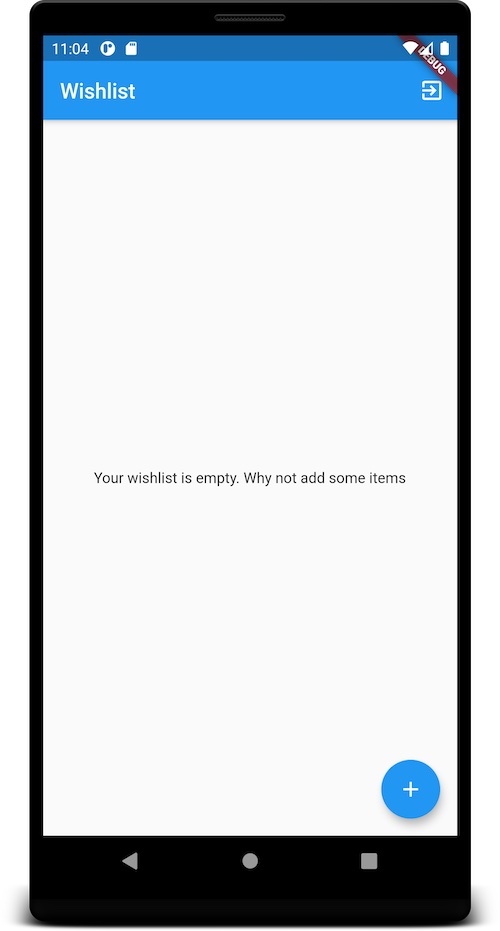This image appears to be a screenshot taken from an Android device. This is evident from the navigation buttons visible at the bottom, which include an arrow for "back," a circle for "home," and a square for "recent apps." The image is designed to resemble the front of a cell phone, complete with bezels and a camera bump at the top, though it is likely a mock-up as there are no visible raised buttons on the sides.

The primary screen displays a mostly white background. At the top, the status bar is blue, followed by a slightly lighter blue banner. This banner contains the word "Wish List" in white text, accompanied by an arrow pointing to the right inside a square icon on the far right side.

Centered on the screen is a message in small black text: "Your wish list is empty. Why not add some items" (notably, there is no punctuation after "items").

At the very bottom of the screen, there is a prominent blue circle featuring a white plus symbol in its center, suggesting an option to add items to the wish list.